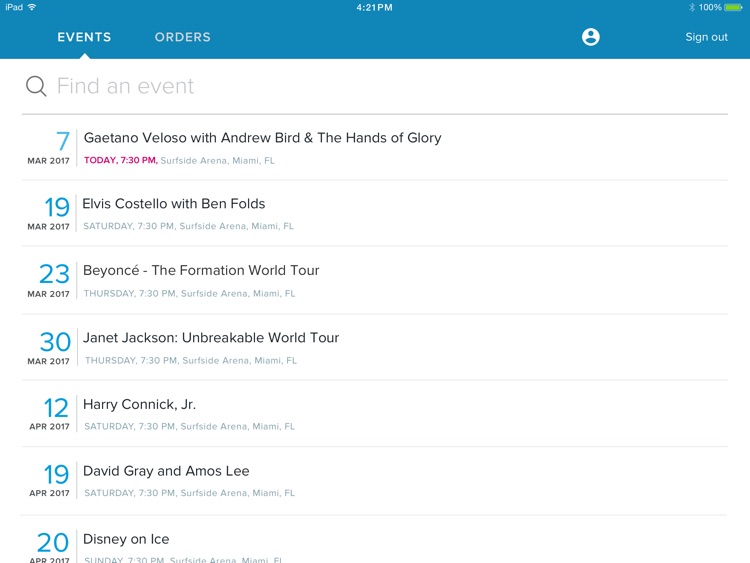This is a vertical image likely captured from someone's iPad screen. The background is primarily white, potentially derived from the device's display. At the top of the screen, there is a thick teal rectangle forming the header. In the upper left-hand corner of this header, the text "iPad" is displayed in white next to the Wi-Fi symbol, both indicating connectivity status. The center of the header shows the time "4:21 PM," while the right-hand side features a Bluetooth icon and a battery indicator at 100% in green.

Beneath this header, there are tabs labeled "Events" (highlighted in white) and "Orders" (in a lighter shade). A generic circular profile picture is positioned on the far right, alongside the "Sign Out" option. Below these tabs, against the white background, lies a search bar with a magnifying glass icon and the placeholder text "Find an Event" in gray. A long gray line acts as a separator, distinguishing this section from the event listings below.

The event listings are organized by date, with the day prominently displayed in blue and the month and year in black. For example, it reads "7 March 2017." The first event listed is "Jayantano Veloso with Andrew Byrd in the Hands of Glory," scheduled for "today at 7:30 PM," highlighted in purple, at the "Surfside Arena, Miami, Florida." This format continues consistently, detailing each event's date, time, and location.